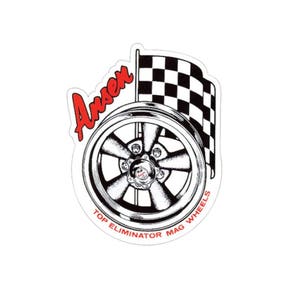The image showcases a cutout sticker or magnet placed against a plain white background. It primarily features a detailed, black and white illustration of a wheel, focusing on the central part without the rubber tire. The wheel has five spindles extending from a central hub, where five lug nuts are visible along with a center circle. Beneath the wheel, the words "Top Eliminator Mag Wheels" are prominently displayed in bold, arching red letters. Enhancing the dynamic design, a black and white checkered flag unfurls behind the wheel, attached to a simple white pole. To the left of this flag and positioned above the wheel, the word "ANSEN" is elegantly written in red cursive letters, emphasizing its brand distinction. The intricate shading in the drawing accentuates its vintage and mechanical allure.